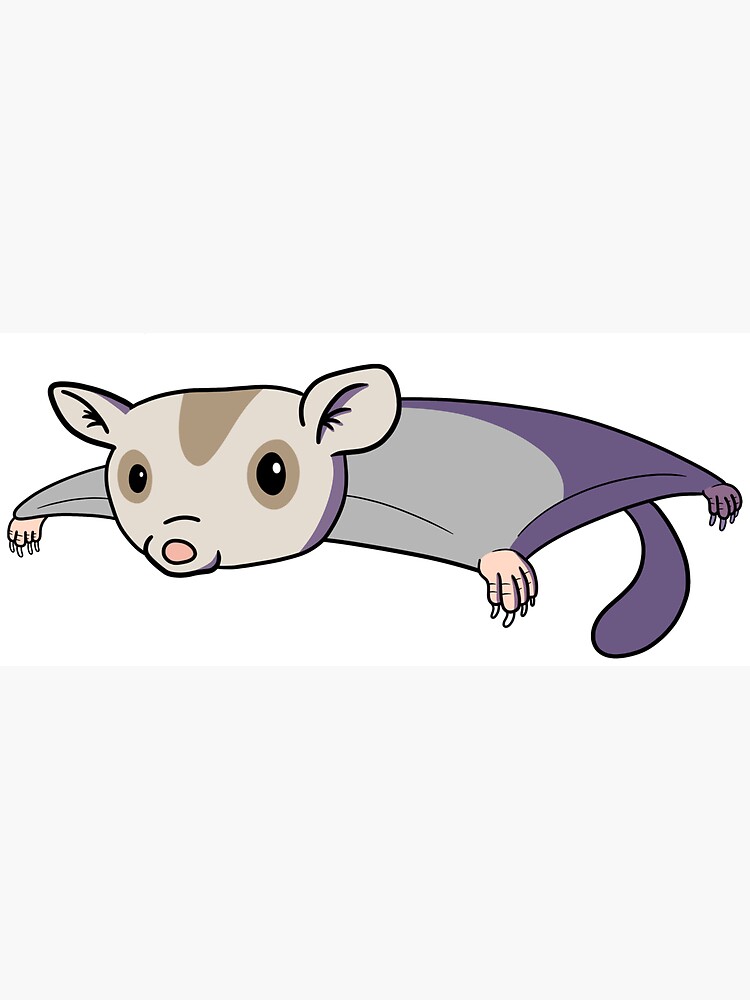The image depicts a simple, cartoon representation of a flying squirrel-like creature, centered on a white background. The squirrel's body starts off as gray, transitioning to a shadowed purple in the lower half. Its head is a light tan-gray with darker tan circles around its brown eyes and a brownish stripe running down the first third of its face, leading to a small, pink nose jutting out. The ears are large and pointy, positioned on the sides of its head. The creature's arms, stretched out as if in mid-flight, reveal a pinkish-tan color, while the back foot visible is shaded purple. The limbs end in fingers with long nails. The tail, shaped like a squirrel's yet lacking fur, resembles a beaver's flat and hairless appendage, emphasizing the two-dimensional nature of the drawing. The overall positioning suggests the flying squirrel is soaring through the air.